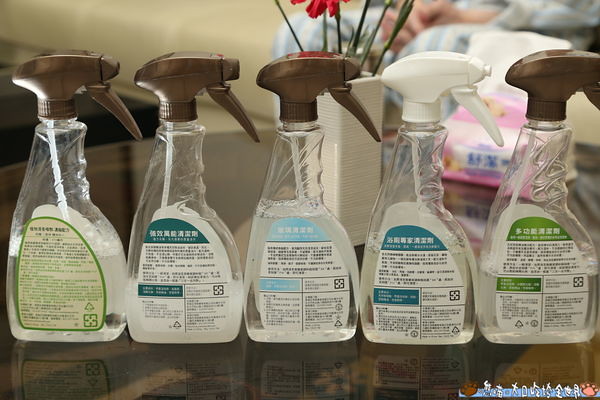This wide-angled color photograph showcases five clear plastic spray bottles, lined up in profile on a glass tabletop. Each bottle contains varying amounts of clear liquid, visible through the transparent containers. The first, second, and third bottles have a copper-colored spray head, while the fourth has a white spray head, and the fifth returns to copper. Detailed labels, adorned with heavy text in a foreign language, decorate each bottle: the first label features light green and cream accents, the second is teal and white, the third is cyan and white, the fourth offers a different shade of teal and white, and the fifth is green and white. Positioned neatly in a row, the bottles obscure their brand names, instead showing their back labels and instructions. An off-white vase with red flower stems and petals peeks from behind the lineup, accompanied by a pink container on the table. In the background, a blurry figure’s hands are faintly visible, adding a human element to the composition.